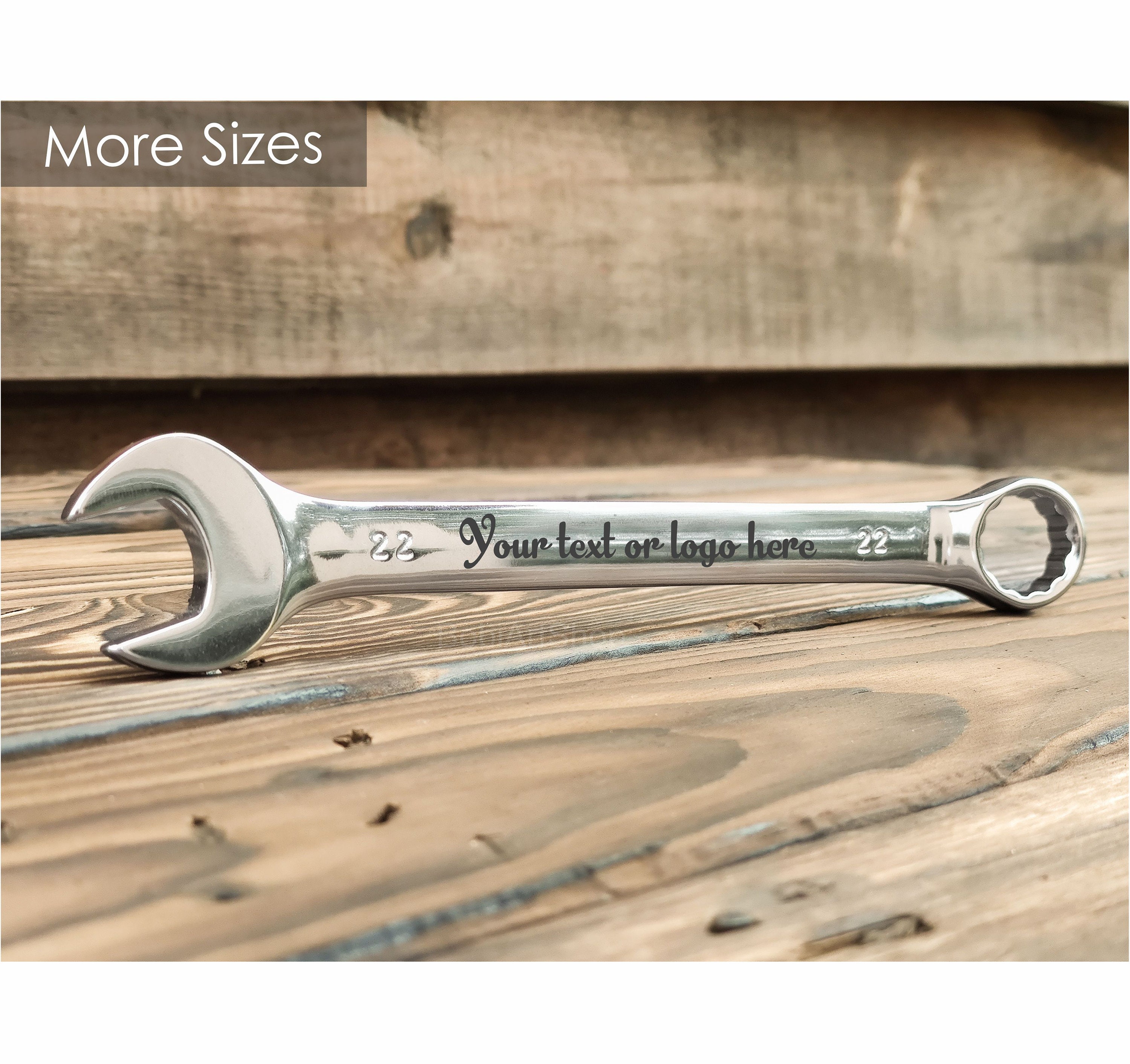In this rectangular photograph, likely intended as an advertisement or product listing, a metallic silver wrench, labeled with the number "22" on both its flat and circular ends, stands upright on its sides against a light-colored wooden surface. The wood beneath it clearly showcases its natural grains and warps, while a matching brown wooden wall serves as the background. The wrench’s sleek, reflective stainless steel surface catches light, casting minimal shadows. Overlay text in stylish fonts adorns the image: a black ribbon in the top-left corner reads "More Sizes" in white, and stretched across the wrench, a bold black text states "Your Text or Logo Here," highlighting its potential for personalization.